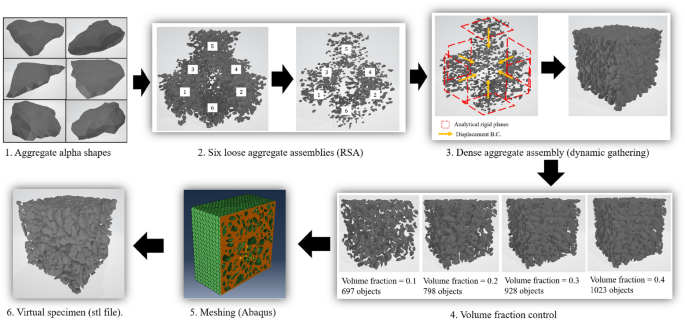The image is a detailed flowchart that appears to be from a science textbook, illustrating the transition of rock formations through various stages of aggregation and assembly. It begins in the top left with a section labeled "1: Aggregate Alpha Shapes," showcasing six images of similar-looking rocks arranged in a 2x3 grid. These lead to step "2: Six Loose Aggregate Assemblies (RSA)," depicted as a formation of smaller rocks labeled from 1 to 6, resembling a loosely structured cluster.

A black arrow moves from this cluster to step "3: Dense Aggregate Assembly (Dynamic Gathering)," where the formations become more compacted, showing a transition from a bush-like structure to a more solid, cubic shape outlined by red squares suggestive of increased density.

Directly below this, step "4: Volume Fraction Control" continues the process. It is divided into four stages, each showing the cubic structure progressively thickening. The stages are annotated with "Volume Fraction" values ranging from 0.1 to 0.4, correlating to an increasing number of objects from 697 to 1023.

On the left of step 4, a colored step "5: Meshing (Abaqus)" presents a green grid resembling a cut geode, with an inner core composed of colorful shapes like a fruit salad, indicating an advanced stage of processing.

Finally, an arrow points to step "6: Virtual Specimen (STL File)," where the cubic formation is rendered in black and white, representing the final digital representation of the specimen.

Overall, the chart visually maps the transformation of rock aggregates from loose assemblies to a dense, controlled structure, ultimately leading to a virtual model.